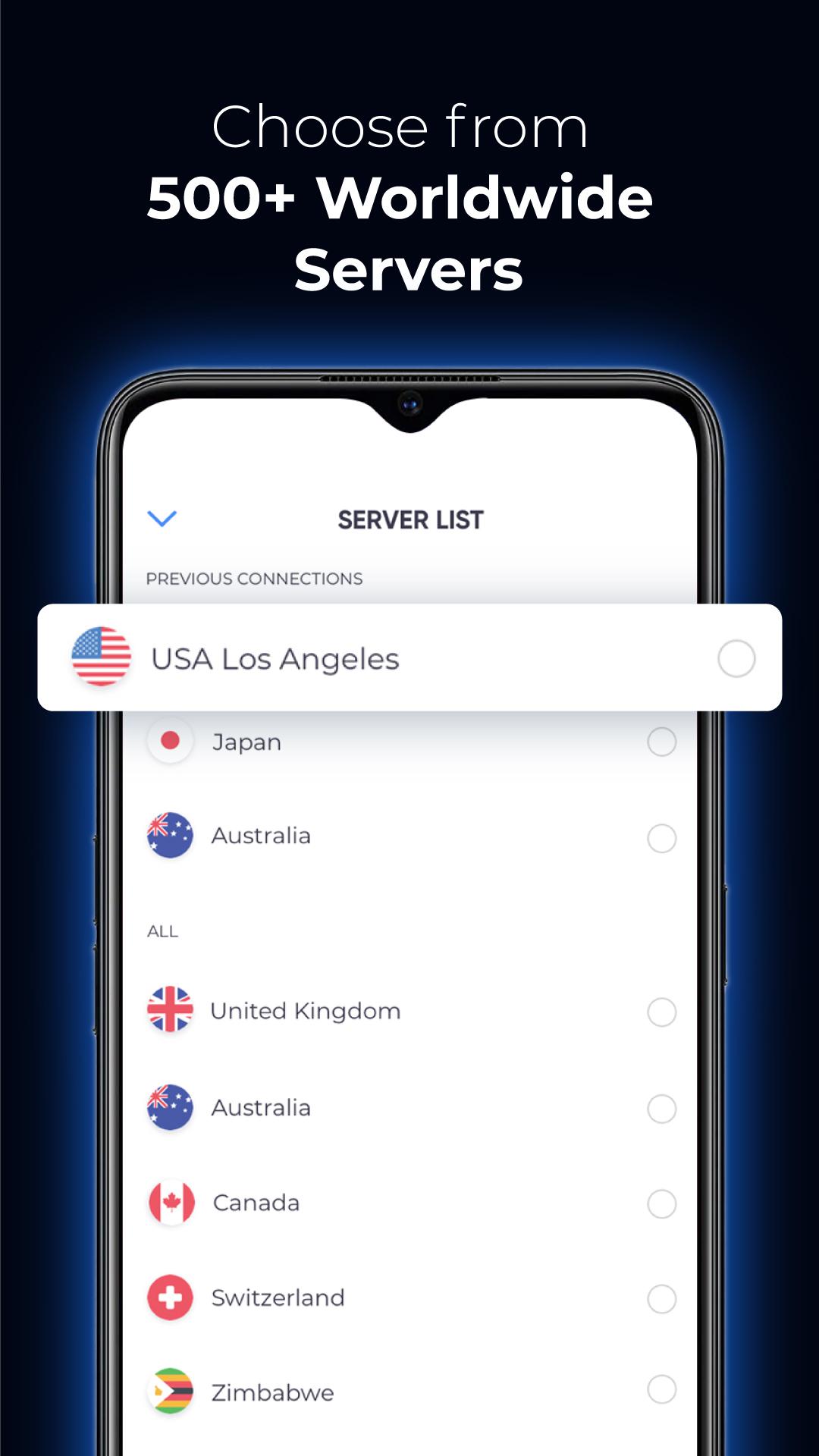The image presents a portrait-mode advertisement with a predominantly black background. At the top, there is white text that reads "Choose from 500+ worldwide servers." Centered below this text is a graphic representation of a mobile phone with a distinctive triangular black notch at the top, likely representing a modern screen design. Surrounding the phone is a subtle blue halo, and it features curved edges, emphasizing a sleek, contemporary look.

On the screen of the mobile phone is a server list displayed on a white page. A prominent blue down arrow indicates the dropdown menu for previous connections. At the top of this list is an entry that appears to extend beyond the confines of the phone screen, labeled "USA Los Angeles" with an accompanying image of the U.S. flag, suggesting it is the selected or highlighted server.

Below this highlighted server, the list continues with various countries and their flags: Japan (Japanese flag), Australia (Australian flag), United Kingdom (UK flag), another entry for Australia, Canada (Canadian flag), Switzerland (Swiss flag), and Zimbabwe (Zimbabwean flag). Each country is represented by a small, round icon of its flag on the left side of the list.

Additionally, there is a placeholder for selecting these servers on the right-hand side of each entry, though none are currently checked. The top of the list features a label for "Previous Connections", reinforcing the Los Angeles server as previously used or favored.

There are no other elements or distractions in the advertisement, keeping the focus on the server selection interface. The minimalistic design underscores the primary message of offering a vast selection of over 500 global servers to choose from.